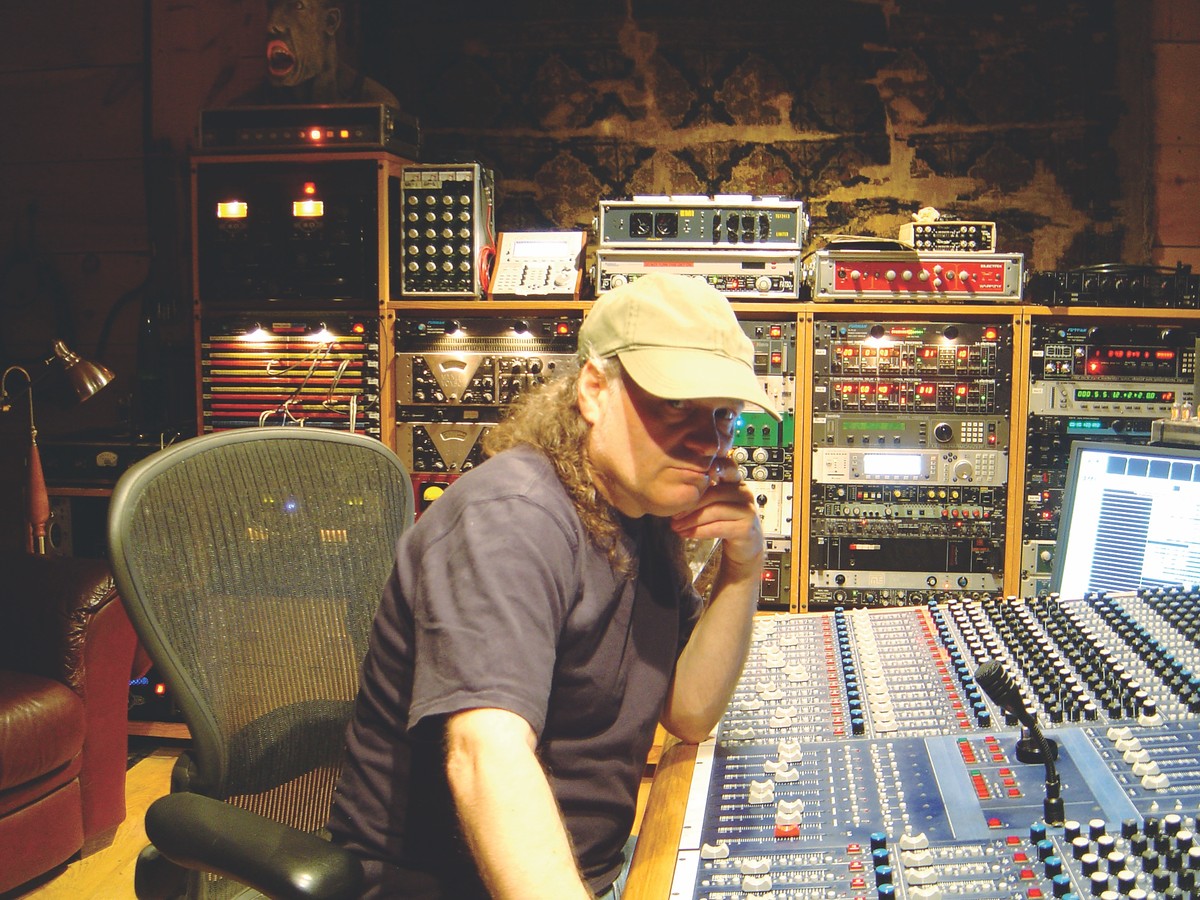This indoor photograph captures a detailed scene in a bustling recording studio, featuring a man as its focal point. Central to the image, the man is leaning forward on a sizable sound mixing console that dominates the right portion of the frame. The console is intricate, brimming with dozens of knobs, dials, and buttons for precise sound adjustments, and includes a microphone for communication with the recording booth. The man, a Caucasian with long brown hair spilling from under a tan baseball cap, wears a blue t-shirt and rests his left elbow on the console's wooden edge. His left hand props up his cheek, projecting an expression of feigned annoyance while he looks directly at the camera, his face partly shaded by his cap. He sits on a black wheeled chair; immediately behind him, a brown leather chair is visible. The recording studio surroundings are dense with stacked equipment housed in wooden shelves, displaying a myriad of lit buttons, joysticks, levers, and screens, all contributing to the high-tech ambiance. A red recliner and a desk lamp are discernible on the far left, adding to the room's eclectic yet organized feel.